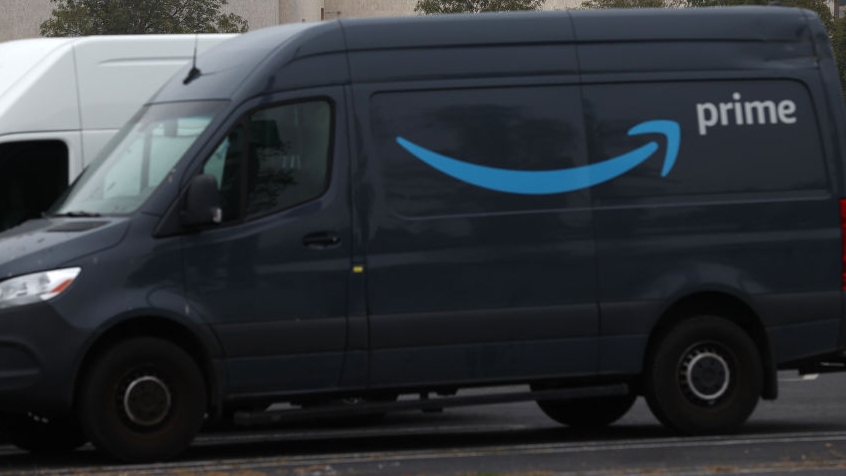A detailed image of an Amazon Prime delivery truck occupies the entire frame. The truck is predominantly blue-black, featuring the unmistakable Amazon Prime branding—a light blue arrow underlining the word "Prime" in bold white text. The vehicle rides on sleek black wheels, and its presence is a familiar sight, depicting the pervasive reality of Amazon's delivery fleet encountered regularly in day-to-day life.